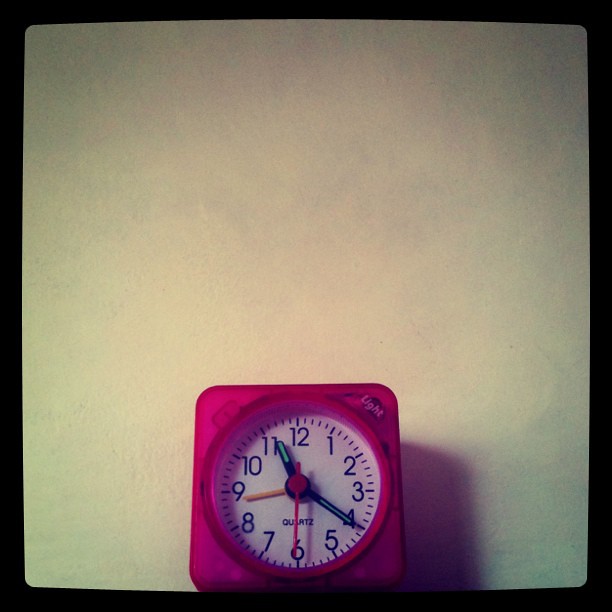The photograph depicts a vibrant and eclectic clock set against a square, black background. The background has subtle gradations, transitioning to gray in the corners, possibly due to lighting effects. The centerpiece is a striking, bright pink lucite clock, semi-translucent in nature, positioned centrally at the bottom of the frame. 

The clock features a circular white face, meticulously marked with numbers from one to twelve, with four small lines demarcating the intervals between each number. The clock hands are distinct and colorful, each serving a specific purpose: a gold hour hand, a black minute hand with hints of green, and a red second hand. There is also a fourth gold hand, likely used for setting the time, suggesting this could function as a small alarm clock.

The clock bears the inscription "QUARTZ" on its face, indicating its mechanism. Additionally, the upper right-hand corner appears to have the words "Light Up," suggesting a potential luminous feature for visibility in the dark. Overall, the photograph captures the essence of a charming, multifaceted timepiece blending practicality with playful design.